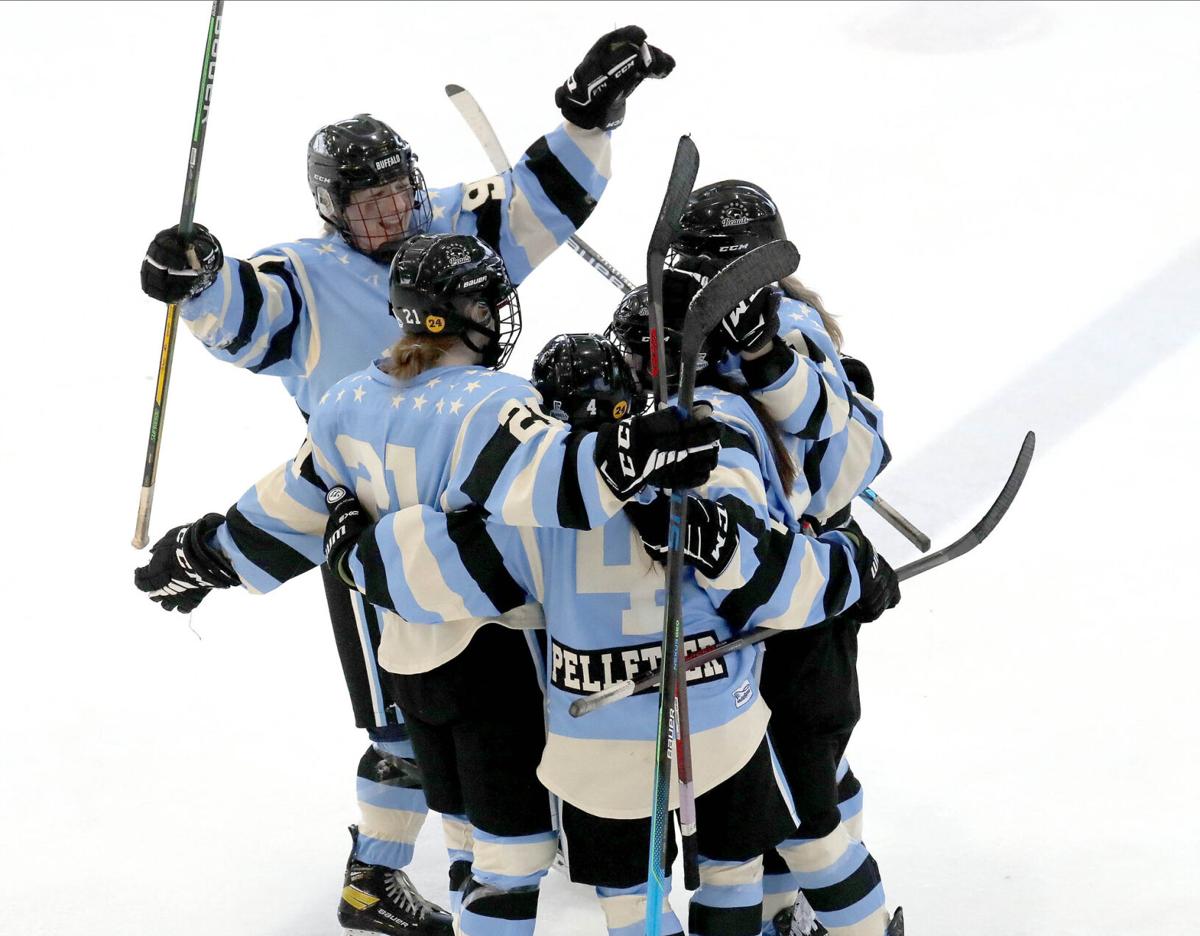In this photograph, a jubilant ice hockey team is captured in the midst of celebration on the ice. Four players are gathered in a close embrace, hugging and visibly elated, while a fifth player stands to the left with both arms raised in triumph, a wide smile on his face, and holding a hockey stick in his left hand. The players are wearing matching uniforms consisting of light blue jerseys with black and white stripes on the sleeves, black shorts with white numbers, and long blue and white striped socks. They are equipped with black helmets and large black gloves and are standing on the ice, clearly overjoyed, perhaps from a recent victory. Visible details include the numbers on their jerseys, such as 21 and 4, and a name that appears to be Peloton or Pelotor.